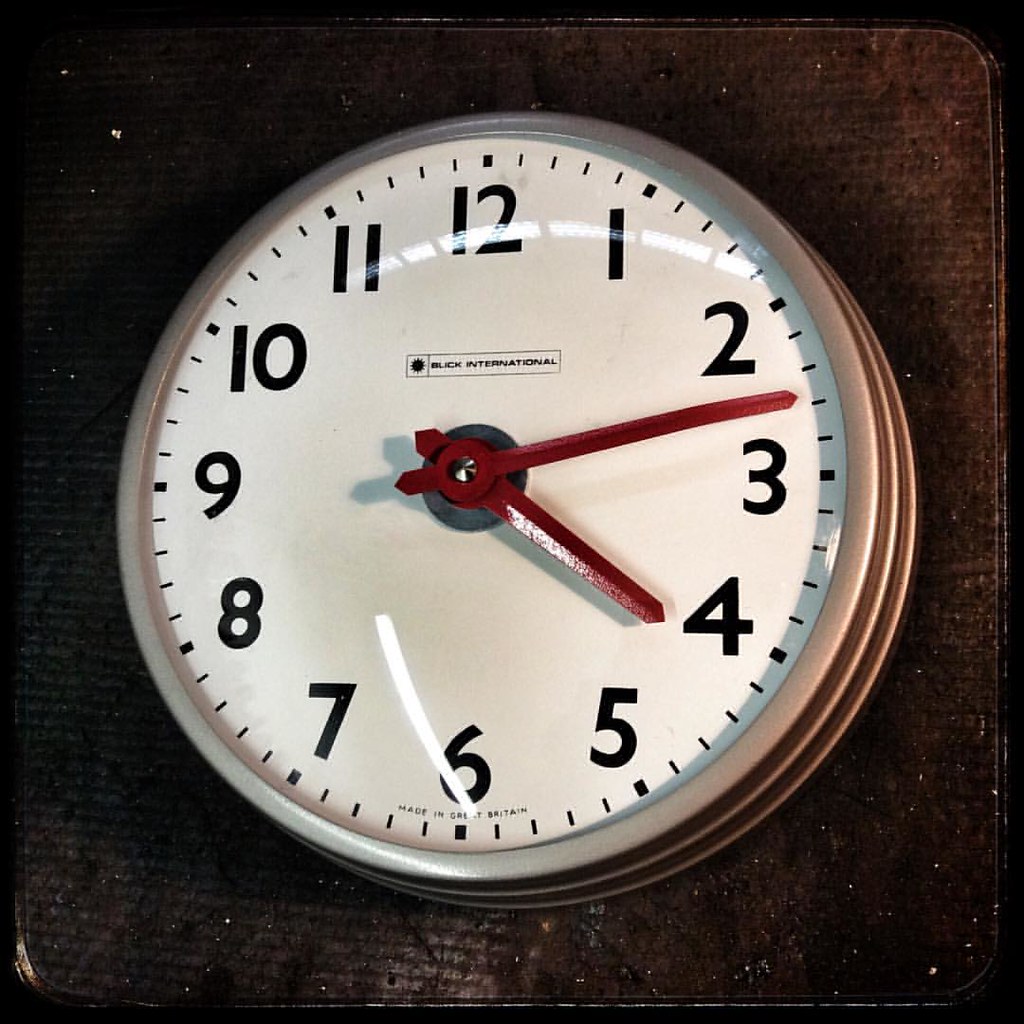This image depicts a color photograph of an analog wall clock mounted on a distressed dark wood background. The wood, aged and worn, features white spots, striations, and markings, particularly on the right side. The clock has a metallic frame with a hue transitioning between silver and copper. Its white face displays black, standard numerals, with minute markers in between, and striking red hands for the hours and minutes. Notably, there is no second hand. Above the center of the clock, "Blick International" is printed in black font, enclosed within a rectangular outline. Below the number six, "Made in Great Britain" is subtly inscribed. The clock's glass covering captures reflections, adding to the details. In the upper right, a corner of the wooden board is rounded, emphasizing the clock against the contrasting dark background.